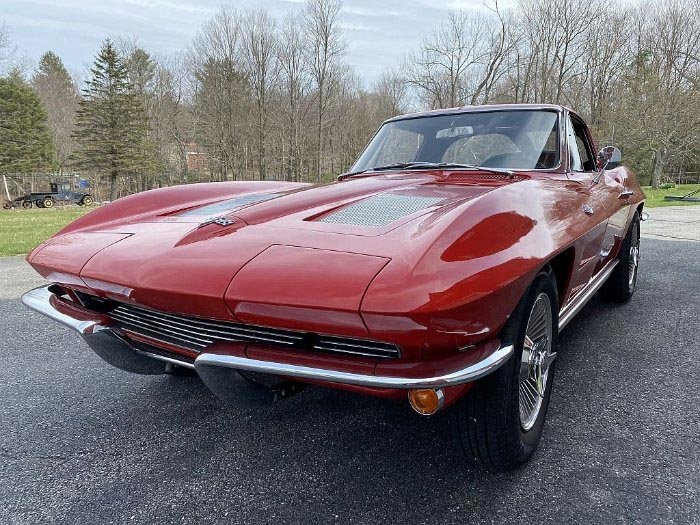This photograph captures a striking, vintage red Corvette prominently positioned in what appears to be a driveway or a secluded side street. The Corvette, a shining example of classic American muscle car design, boasts a lustrous, cherry candy red finish accented by chrome features. The front of the car displays a distinctive chrome push bar with a curved shape, along with a black grille adorned with white lines. The hood is notable for its mesh-like panels on either side of the Corvette's emblem, and the car is further complemented by its black wheels with silver rims. 

Viewed from a corner angle, the image draws attention to the car's sleek, streamlined body and coupe design, revealing a single door handle and the curvaceous contours of this two-door sports car. In the background, the scene is set against an overcast, cloudy sky, with bare, leafless trees creating a stark, wintry backdrop. To the left, an old, blue work truck, reminiscent of the 1920s, contrasts with the modern elegance of the Corvette. The setting is quiet and spacious, with the car parked on a dark gray, paved driveway, enhancing the timeless appeal of this meticulously maintained classic vehicle.